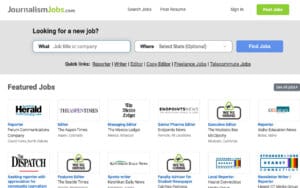This image depicts a grainy and slightly blurry webpage with a predominantly white background and black text, interspersed with some blue highlights. The webpage is identified as journalismjobs.com, with the logo styled such that "journalism" appears in grey and "jobs" in green. In the top left corner, the website name is clearly visible.

Along the top of the page, there are multiple tabs, although they are not clearly readable. However, a grey sign-in button and a green login button are discernible on the top right. The main content of the page features a job search section. On the left side, there is a prompt that reads "Looking for a new job," accompanied by a filter option to sort by job type. Directly to the right, a prominent blue button labeled "Find Job" stands out. Below this section, additional tabs are present, though they are unfortunately unreadable.

Towards the bottom left of the image, there is a section titled "Featured Jobs," showcasing a list of job opportunities. Out of the ten featured positions, only two are legible: one from the Herald and another from the Dispatch. The remaining job listings are less clear, with grey text that is difficult to read.